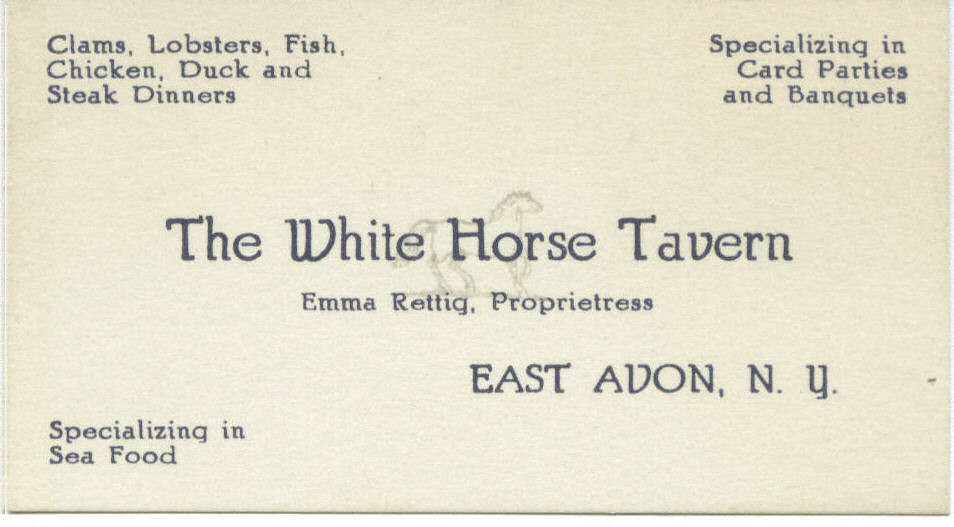The image features a vintage, cream-colored business card for the White Horse Tavern, located in East Avon, New York. At the center of the card, in large, prominent text, is the name "White Horse Tavern," with a subtle, faint graphic of a horse behind the text. Directly below the establishment's name, it lists "Emma Rettig, proprietress." The card appears slightly worn, indicating its age. On the top left, there's a list of food offerings: clams, lobsters, fish, chicken, duck, and steak dinners. Across from this, on the top right, the card highlights the tavern's specialty in card parties and banquets. Additionally, the bottom left corner mentions "specializing in seafood" in a similar font style. This card serves as a detailed promotional piece for the tavern, enticing potential patrons with its diverse menu and event hosting capabilities.